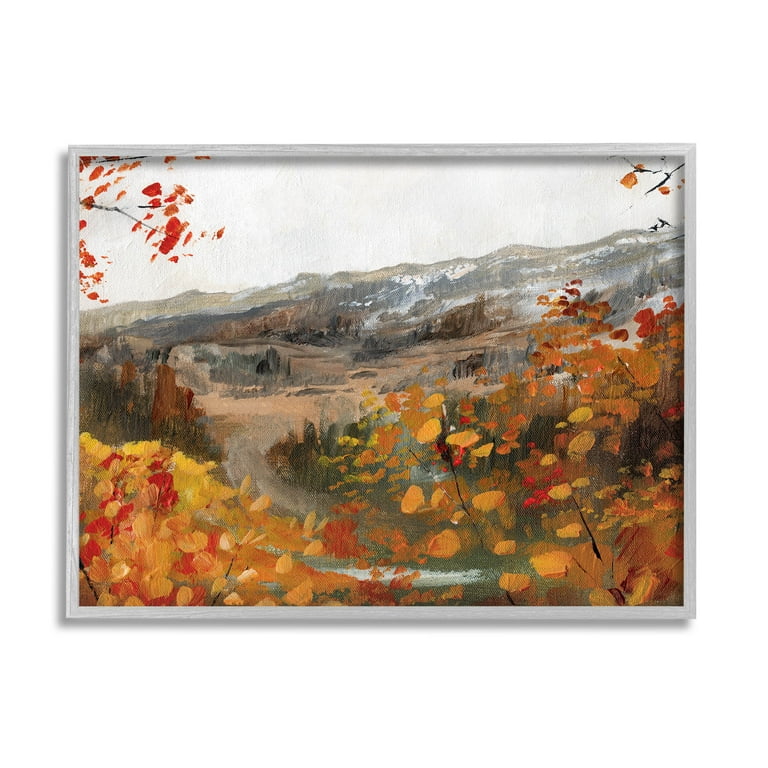This is a photograph of a framed impressionist oil painting capturing an autumnal mountain and forest scene. Encased in a simple, almost silvery grey to white wooden frame, the painting is characterized by rough, large brush strokes that evoke the essence of a fall landscape. The foreground is dominated by vibrant reds, oranges, and yellows of leaves and bushes, with suggestive blobs of color rather than detailed shapes. Through the branches and leaves that arch into the scene from the upper corners, you can glimpse a path lined by trees that guides the eye towards gently sloping hills and rugged mountains dusted with snow. The background reveals a hazy, soft-lit sky in a white or grey hue, enhancing the impression of an overcast day. There is an implied presence of a waterway or stream weaving through the scene, with random foliage in green and urban orange adding complexity to the view. The entire composition exudes the serenity of an autumn afternoon, where the abstract rendering of nature invites the viewer to wander through this tranquil, yet vivid, landscape.